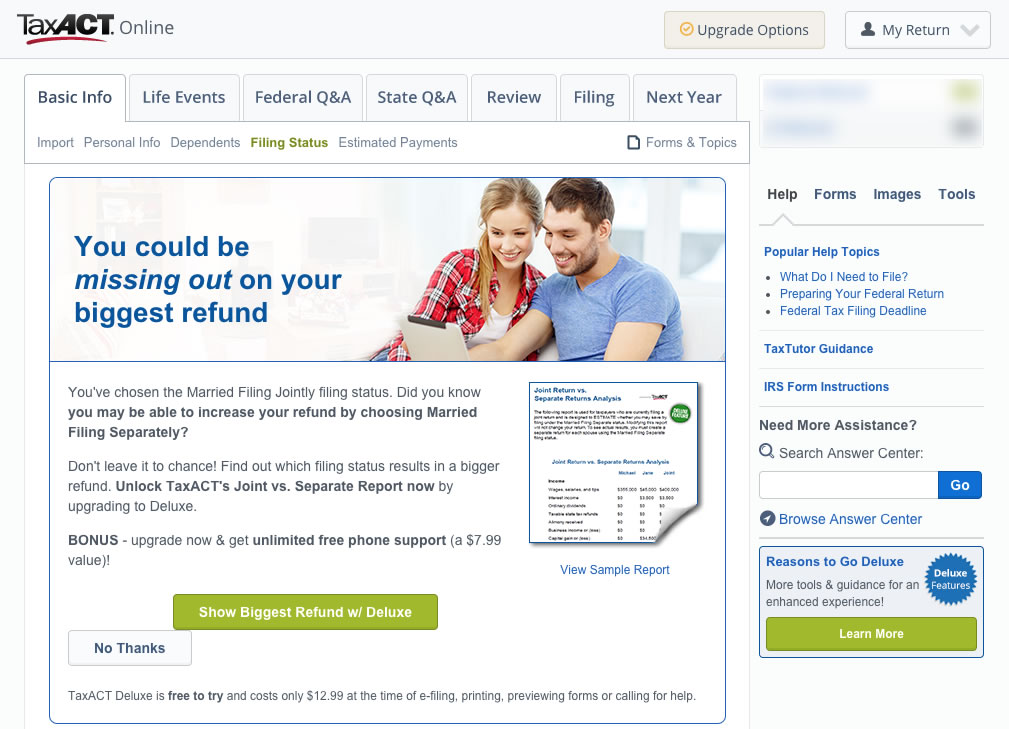The background of this image features a gradient in shades of gray. On the top right-hand side, "Tass Active" is prominently displayed in bold black font with a red underline, followed by the word "Online." 

Beneath this, on the right, are two rectangular boxes. The first box is beige with an orange circular icon that has an orange checkmark; the border of the checkmark is also orange. This box is titled "Upgrade Options" in black text. The second box is white, matching the overall background, and contains the text "My Return" in black.

Below these boxes are several tabs. The first tab, "Basic Info," has a white background. Subsequent tabs include "Import Personal Info," "Dependents," and "Filing Status," with the latter highlighted in yellow. Additional tabs listed are "Estimated Payments," "Forms," and "Topics." 

Another set of tabs have a matching gray color as the primary background and include "Life Events," "Federal Q&A," "State Q&A," "Review," "Balance," and "Next Year."

An image shows a couple looking at a white clipboard. On the left side of this image, there's blue text stating, "You'll be missing out on your biggest refund." Below this, it reads, "Bonus Upgrade Now and get unlimited free phone support" in the same blue color. A green box contains the text, "Show Biggest Refund with Deluxe," and there is an adjacent option labeled "No Thanks."